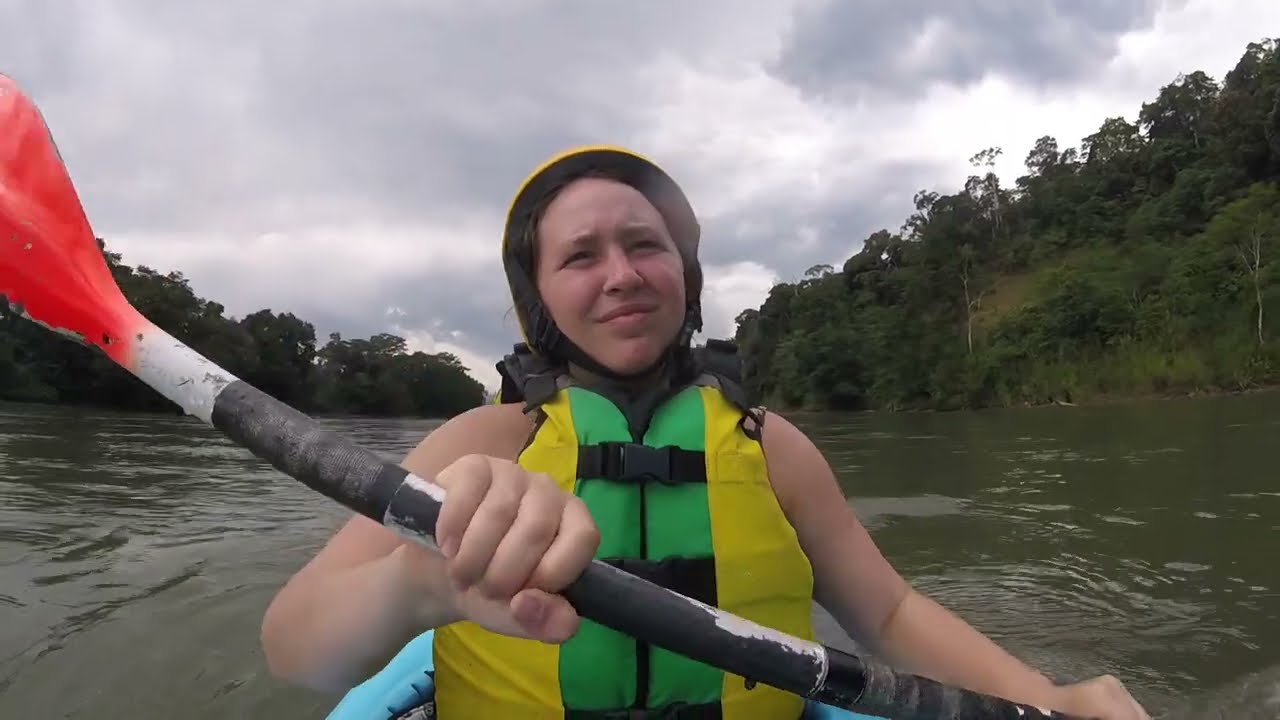The photograph captures a close-up view of a white-skinned woman kayaking in a remote and serene area. She is seated in a blue kayak with her green and yellow lifejacket prominently displayed. Her safety helmet, which is yellow with a black border, conceals her hair, presumably pulled back and tucked inside. She grips a black and white oar with both hands, the orange-red paddle tip visible towards the top left of the image. The scene around her features a river with greenish water and banks lined with dense, deciduous trees. The sky above is layered with white and gray clouds, hinting at the possibility of imminent rain. There are no other people or buildings in sight, emphasizing the natural and secluded environment.